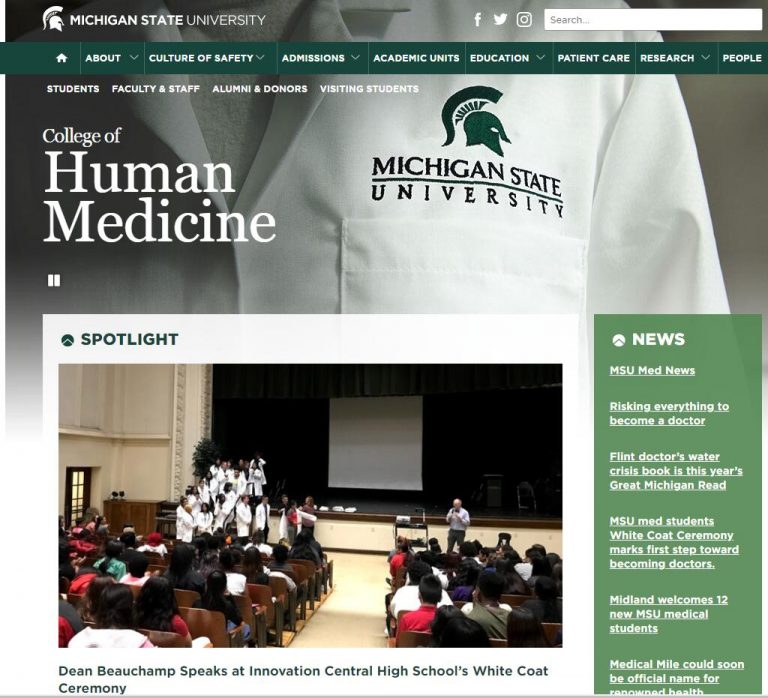The website for Michigan State University's College of Human Medicine features a detailed and thoughtfully designed interface. 

In the top left corner, the recognizable Spartan helmet logo and the name "Michigan State University" are prominently displayed. To the right at the top of the page, social media icons for Facebook, Instagram, and the newly rebranded X (formerly Twitter), are aligned, providing quick access to their respective platforms. Adjacent to these icons is a white search bar, easily identifiable by the gray word "search" inside it.

A green horizontal navigation bar spans the width of the site, serving as the main hub for exploring the website's various sections through its drop-down menus. Just below this bar, four key categories are neatly arranged in white font: "Students," "Faculty & Staff," "Alumni & Donors," and "Visiting Students," offering pathways to more specific information.

Dominating the center of the page is the title "College of Human Medicine," also in white font, which stands out against the background image of an individual dressed in a white doctor's lab coat, emphasizing the institution's medical focus.